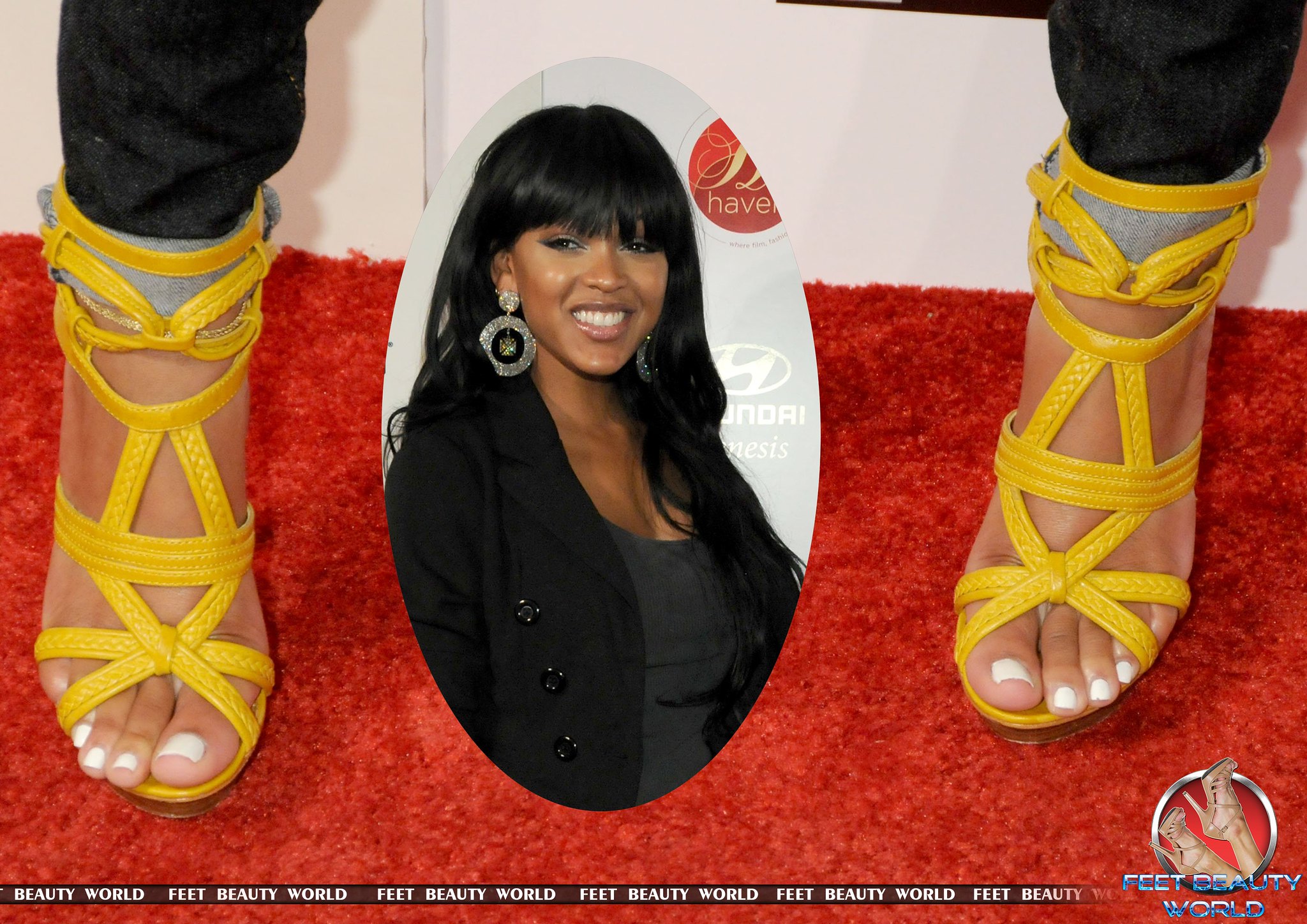The image features a complex overlay of two photographs: an oval-shaped, head-to-torso portrait of a woman superimposed on a background image of feet. The woman has long black hair with bangs, is wearing large circular earrings, a gray shirt or dress, and a black jacket or blazer with buttons, and she is smiling, her makeup immaculate. She appears to be at a red carpet event, where a red carpet and a white screen are present in the background. The second photograph shows someone’s feet adorned in open, strappy sandals, revealing white-painted nails, with long denim pants. Repeated text along a thin banner at the bottom reads “beauty world feet.” Also present is a circle logo with a silver border and red inner section featuring two feet pointed upwards and blue text below that reads "feet beauty world." The image showcases a diverse color palette, including black, white, yellow, red, brown, silver, gray, and off-white.